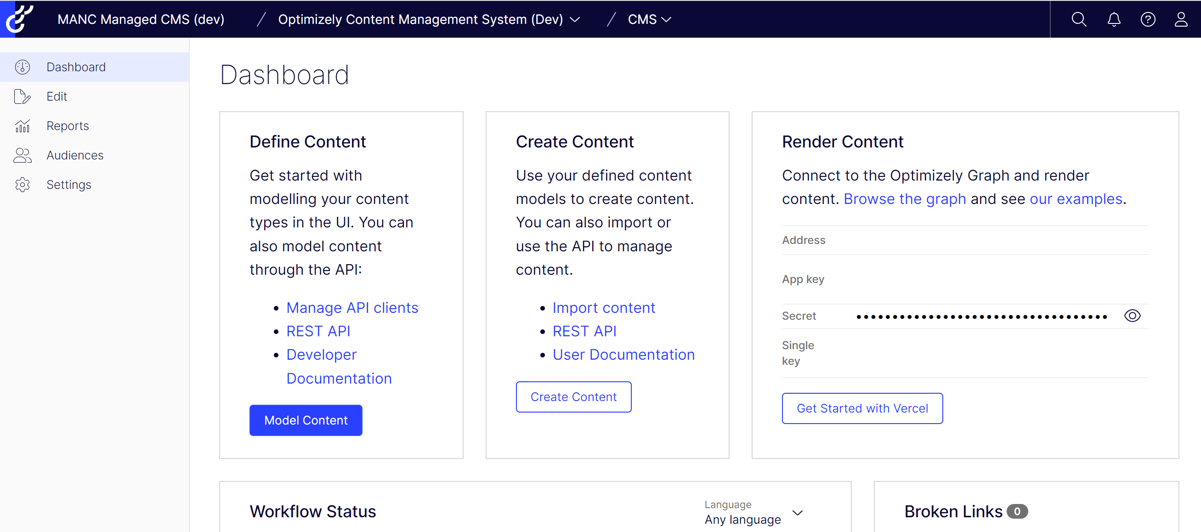**Detailed Caption for the Screenshot of the MANC Managed CMS Dashboard (DEV)**

This image captures a detailed screenshot of the MANC Managed CMS dashboard, specifically for developers, as indicated by the "D-E-V" in parentheses. The dashboard interface appears to be designed with a sleek, black text box featuring white lettering prominently displaying the title "Optimizely Content Management System" with "developer" in parentheses, followed by "CMS" after a slash. 

On the far-right side of the header, there are several icons: a magnifying glass symbolizing search functionality, a notifications icon, a question mark inside a circle indicating help or support, and a user icon for profile or account settings. 

Adjacent to the "MANC" label on the left side is an icon resembling a half-circle with three additional smaller half-circles emerging from it. Below this, the background transitions to gray, where the word "Dashboard" is displayed in black text, enclosed within a light blue text box. Accompanying this section is a dropdown arrow icon.

Further down, the interface presents several menu options:
- "Edit" accompanied by a paper and pencil icon
- "Reports" with a graph icon
- "Audiences" represented by two user icons
- "Settings" depicted with a gear icon

The main content area beneath these menus is split into three sections:
1. **First Box: Define Content**
   - Description: "Get started with modeling your content types in the UI. You can also model content through the API."
   - Bullet Points in Blue Text: Manage API clients, REST API, Developer documentation
   - A blue button labeled "Model Content" with white text

2. **Second Box: Create Content**
   - Description: "Use your defined content models to create content. You can also import or use the API to manage content."
   - Bullet Points in Blue Text: Import content, REST API, User documentation
   - A button outlined in blue with blue text: "Create Content"

3. **Third Box: Render Content** (larger than the first two)
   - Description: "Content to the optimize graph and render content."
   - Features in Blue Text: Browse the graph, and see examples.
   - Examples: "Address, app key, secret" (password hidden with dots), and "Single key"
   - A blue-outlined white box labeled "Get Started with Vercel."

Below these boxes, additional sections include:
- Workflow Status with a top outline
- Language selection dropdown showing "any language" with an arrow for more options
- A scrollable section for Broken Links displaying a "0" inside a black oval

Each of these features is methodically placed to promote a comprehensive and user-friendly developer experience within the MANC Managed CMS.